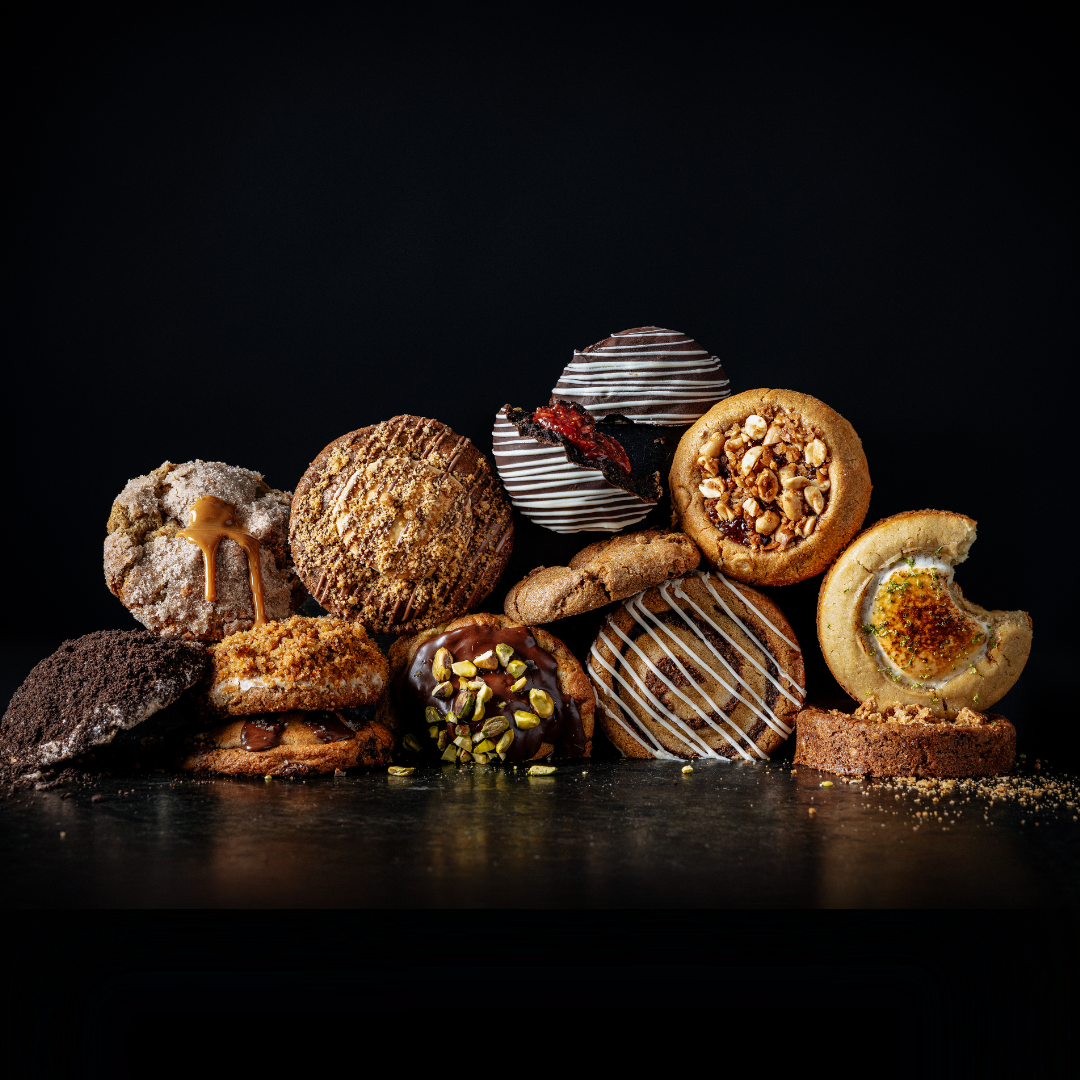This color photograph showcases an assortment of round pastries and cookies meticulously arranged on a glossy black surface with a seamless black background. The high-contrast lighting casts attention solely on the dozen or so baked treats, also creating slight reflections on the shiny base. Among these goodies, you can spot pastries adorned with rich toppings: a cinnamon roll drizzled with white frosting, a muffin-like pastry with caramel oozing over its top, and a cookie sprinkled with brown sugar. Some cookies feature vibrant details, such as a chocolate-coated one with white stripes and a possible red filling at the center, while another displays nuts embedded in its dark chocolate topping. A delicate cookie with brown sprinkles and another with a sugary dusting and caramel highlight the diversity. There are also pastries incorporating nuts like pistachios. Altogether, these treats form a visually inviting mountain of baked goods.